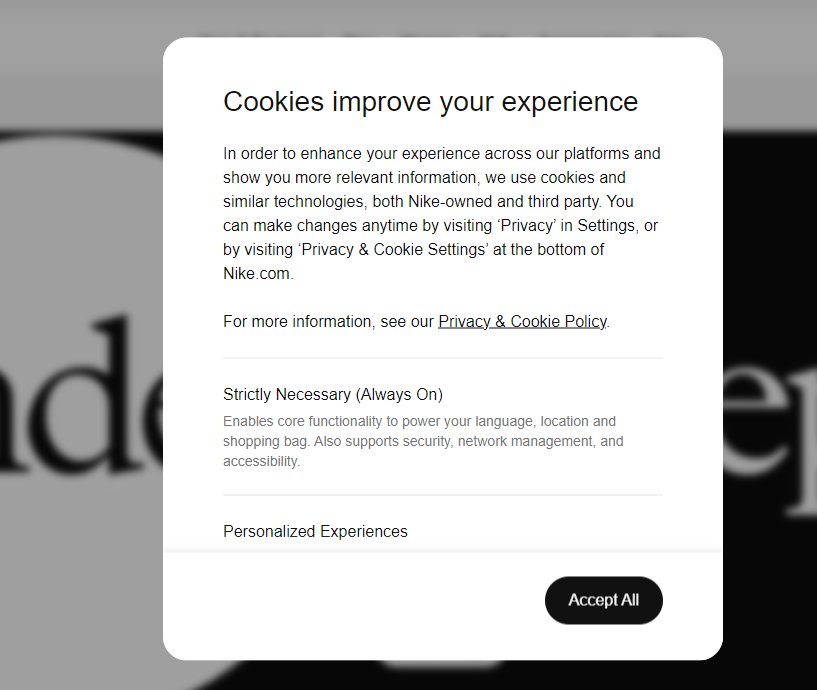The image displays a pop-up dialog box on a website, designed with a sleek, modern aesthetic. The box itself is white with rounded corners. At the top, large black text reads, "Cookies improve your experience." Below this header, a detailed paragraph explains, "In order to enhance your experience across our platforms and show you more relevant information, we use cookies and similar technologies, both Nike-owned and third-party. You can make changes anytime by visiting privacy and settings or by visiting privacy and cookie settings at the bottom of nike.com. For more information, see our privacy and cookie policy." The phrase "privacy and cookie policy" is underlined, indicating it’s a clickable link.

Beneath the paragraph is a light gray bar followed by another section titled "Strictly necessary (always on)." This grey text block states, "Enables core functionality to power your language, location, and shopping bag. Also supports security, network management, and accessibility."

A horizontal gray line separates this section from the next one, which is headed in black text, "Personalized experiences." Another gray line is present in this area, maintaining the visual structure of the pop-up.

At the bottom right of the box is a prominent black, oval-shaped button with the text "Accept All" in white, inviting users to consent to all cookies.

In the background, the webpage appears blurred, with visible areas: a white section on the left with black text, and a black section on the right with white text, maintaining a consistent color scheme and visual hierarchy.